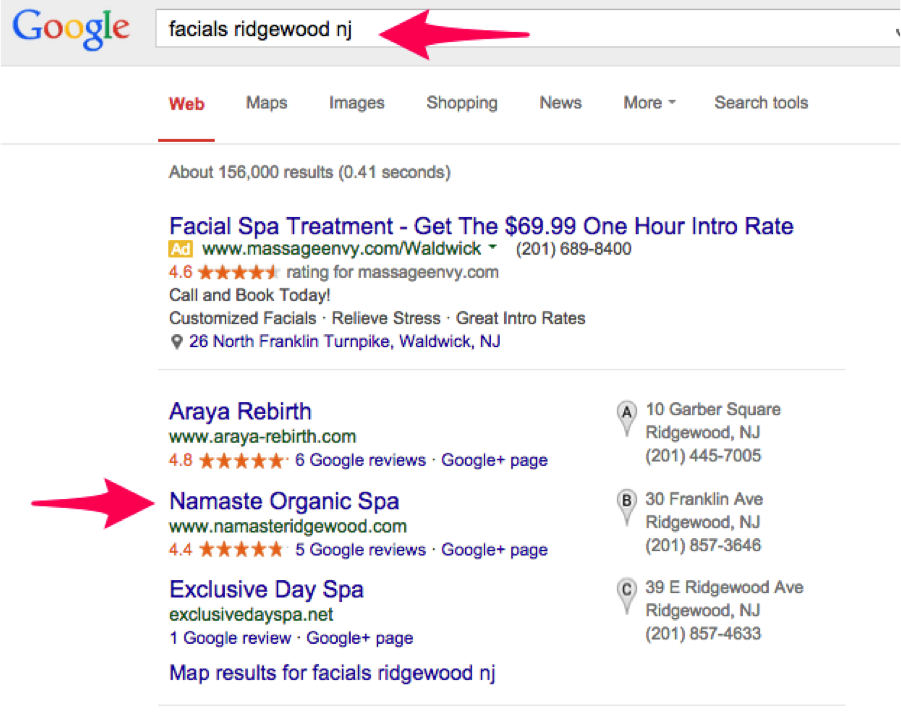The image depicts a Google search results page. At the top, there is a light gray banner with the Google logo in its familiar primary colors. Below the logo sits the search bar containing the query "Facials Ridgewood, New Jersey," highlighted by a pinkish-red arrow pointing towards it.

Beneath the search bar, there is a white background area displaying several search options. In pinkish-red underlined text, it reads "Web," followed by gray text options: "Maps," "Images," "Shopping," "News," "More," along with a drop-down menu and "Search Tools."

The search results indicate approximately 156,000 results, retrieved in 0.41 seconds. The first result is an advertisement for a facial spa treatment offering a $69.99 one-hour introductory rate. The ad includes the business rating, phone number, and a call-to-action to book. 

Further down, the search results list "Array of Rebirth," featuring its address, website, and star rating. Lastly, "Namaste Organic Spa," highlighted by another pinkish-red arrow on the left, is noted with its exclusive day spa services, address, and phone number.